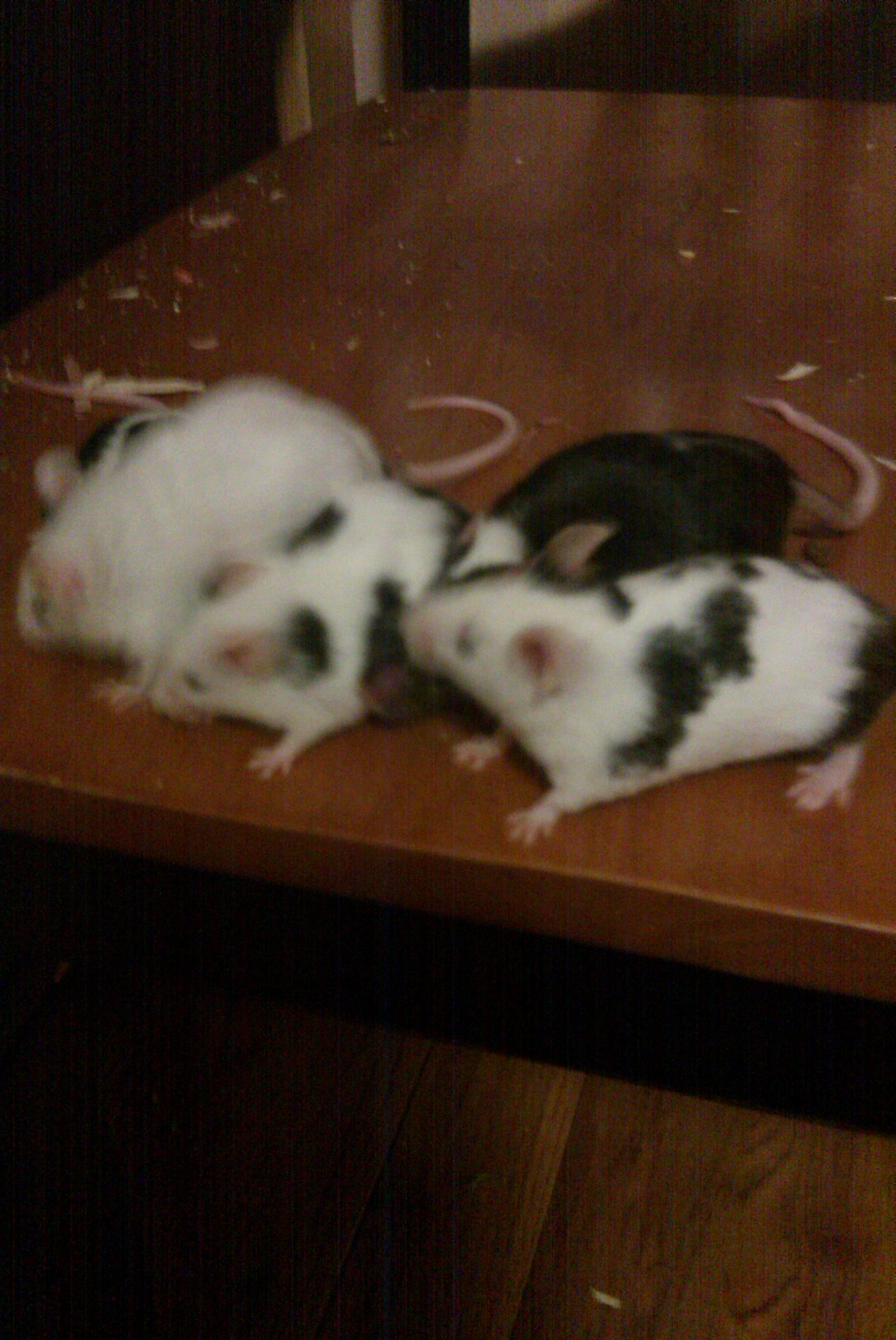This is a slightly blurry photograph of four mice on a dark brown wooden table. The focus is primarily on the background, which is sharp and reveals the detailed wood grain of the table, along with small wooden pellets and dust, indicating the mice have been active. In the foreground, out of focus, are the mice:

1. A completely white mouse with a long pink tail.
2. A black mouse with a white spot on its head.
3. Two mice with a mix of black and white patterns – one predominantly white with black spots and the other primarily black with white patches. 

All the mice have black eyes and little pink feet and seem to be looking towards the left side of the image, slightly facing the camera. There might be an additional, mostly black mouse partially visible on the far left, showing only its head and ears. The cluttered background with wood pellets adds context to the habitat-like setting.